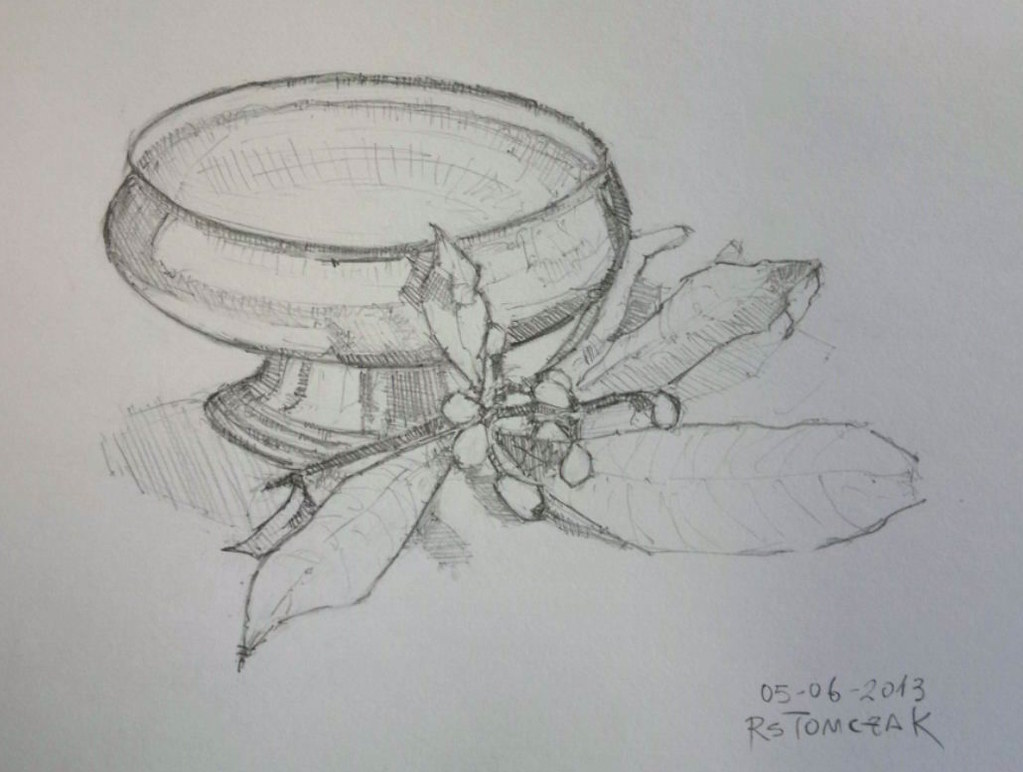This detailed pencil sketch is rendered on a textured white cardstock paper and prominently features a large, shallow bowl or chalice. The bowl has a wide, expansive opening, similar to a wine glass but more substantial in width, supported by a pedestal that narrows in the middle and flares out at the base, adorned with three concentric rings. In the foreground, a sprig of plant life, possibly mistletoe or poinsettia, lies gracefully beside the bowl. This plant includes a dark-colored stem, several intricately textured, jagged oval-shaped leaves, and clusters of small berries. The entire drawing, done solely in black pencil with attention to shading and detail, occupies the majority of the upper left space of the frame. The sketch is signed and dated in the lower right corner with the inscription "05-06-2013 R.S. Tom C.Z.A.K."